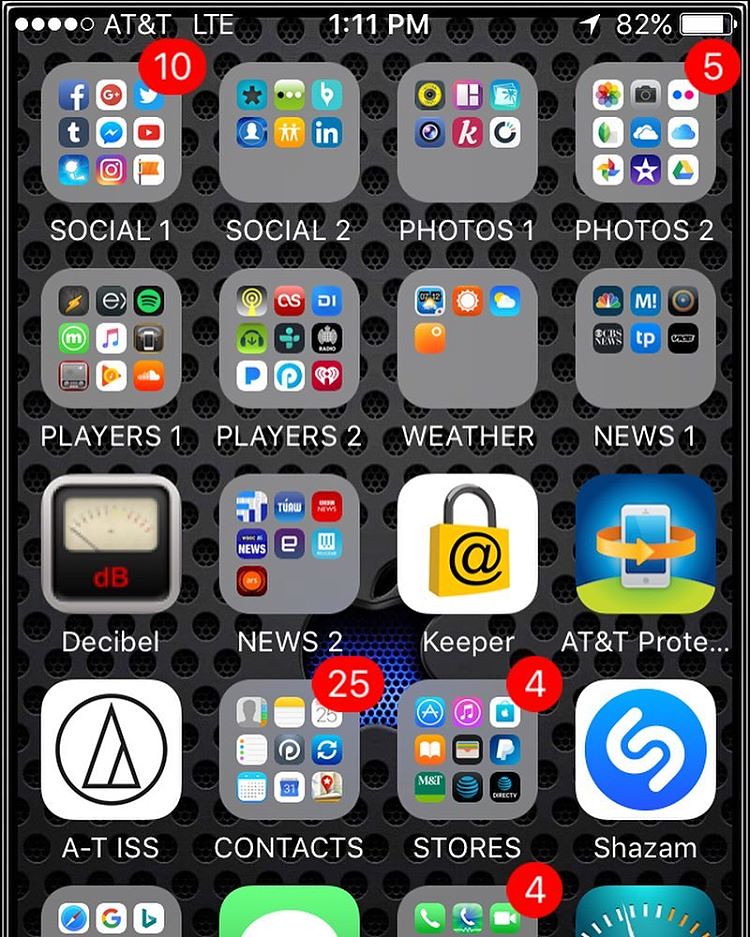This is a detailed screenshot of a smartphone's home screen. The display is framed by a grayish perimeter, highlighting the central area filled with distinct app icons. Each icon is square with rounded edges, systematically arranged in rows of four, presenting a structured yet colorful grid.

At the top, the first eight icons are miscellaneous collections grouped under the labels: Social 1, Social 2, Photos 1, Photos 2, Players 1, Players 2, Weather, and News 1. Social 1 is notable for a red circular notification badge displaying the number 10, while Photos 2 has a similar red circle with the number 5.

Underneath this top row, there are individual app icons including:
- Decibel: Featuring a small black device with a gauge, suggesting an audio measurement tool.
- News 2: Another app bundle.
- Keeper: Distinctive with a yellow lock and an '@' symbol, indicating a password manager or security app.
- AT&T Protect: Showcases a phone icon wrapped with an orange ribbon, hinting at a protection or insurance service.
- AT&T ISS: Displayed with a white background and a triangle within a lined circle, suggesting a security or identity service.
- Contacts: Essential utility presented with a standard icon design.
- Stores: Similarly styled, representing app or media stores.

Finally, near the bottom edge of the screen, part of additional app icons are visible, including Shazam - a blue circle with two curved white shapes reminiscent of a music discovery service.

Overall, the screenshot encapsulates a variety of applications, each with unique visual identifiers and some with active notifications, suggesting a frequently used and organized smartphone interface.